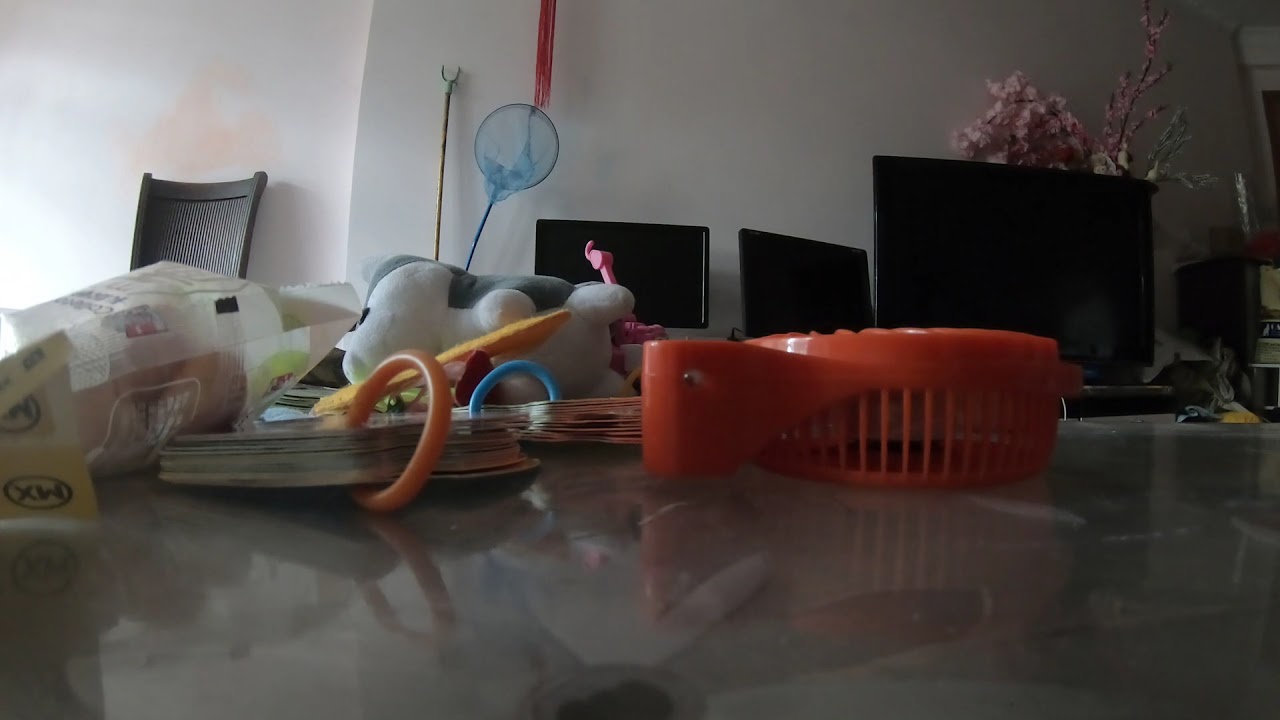The image depicts an eclectic indoor scene featuring a variety of household and personal items, likely set in someone’s living room or kitchen during the day. In the foreground, atop a glass-topped or slate table with a floral print, several objects are prominently displayed. These include a bag of snacks possibly containing a soda can, various children’s toys, a gray and white stuffed animal, two ring-bound flip books, and a bright orange handheld fan. The table is positioned centrally, reflecting some of the items upon it.

In the midground and background of the image, the scene expands into a broader view of the room. To the left, an orange stain marks a white wall beside which a brown chair is leaned. Adjacent to this is a pole and a blue pool-skimming net. Further into the background, three dark computer monitors—two medium-sized and one larger—are visible, flanked by a pink flower and additional unidentifiable garden objects. Despite the varied assortment of items, there is no visible text within the image. The color palette includes hues of white, pink, gray, light blue, black, orange, and yellow, contributing to the detailed and somewhat cluttered atmosphere.